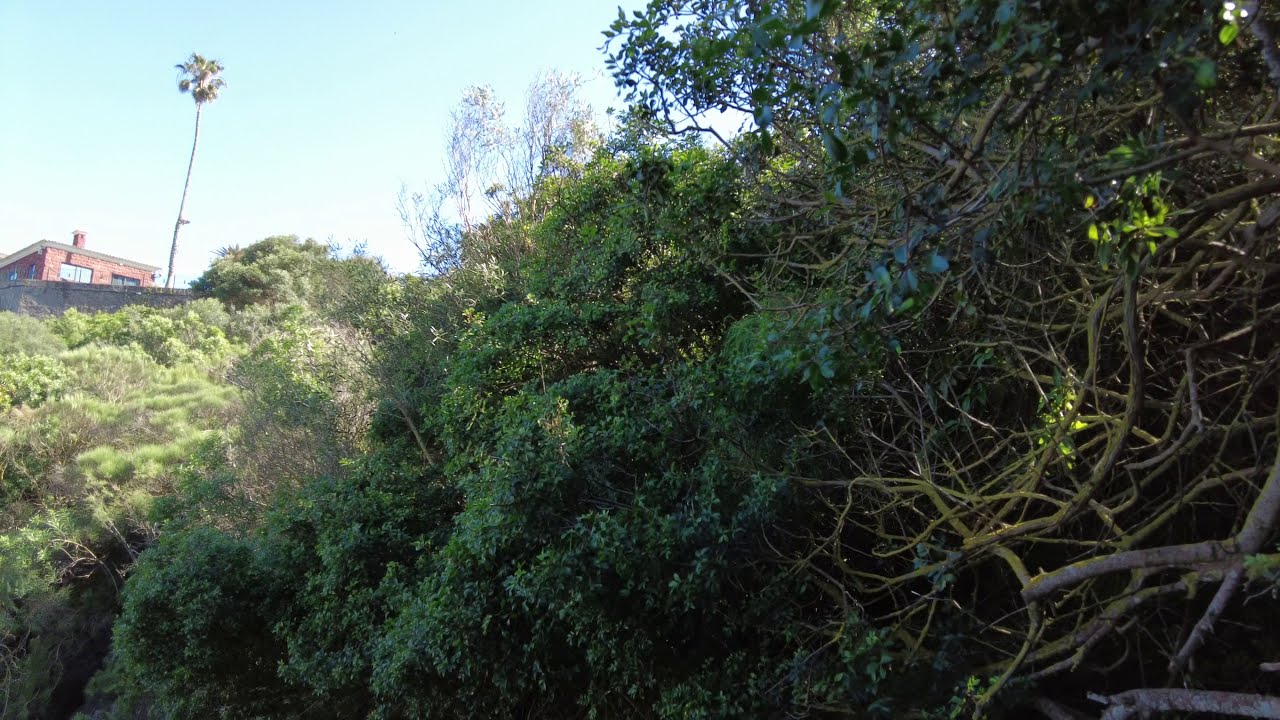The photograph depicts a sunlit outdoor scene taken from the bottom of a ravine or a small valley. Dominating the right side of the image are thick brambles and bushes with dense, leafy green foliage interspersed with dark branches. The vegetation appears to form a dense thicket that stretches from the top right of the photo to the lower left corner. On the left side of the photograph, a red brick building with a flat roof and a chimney stands behind a wooden fence. A tall, slender palm tree with fronds at the top rises next to the building. The background reveals a clear blue sky, contributing to the bright and sunny ambiance of the scene. The contrast between the illuminated greenery on the downslope of the hill and the shadowed foliage to the right enhances the depth and texture of the landscape.